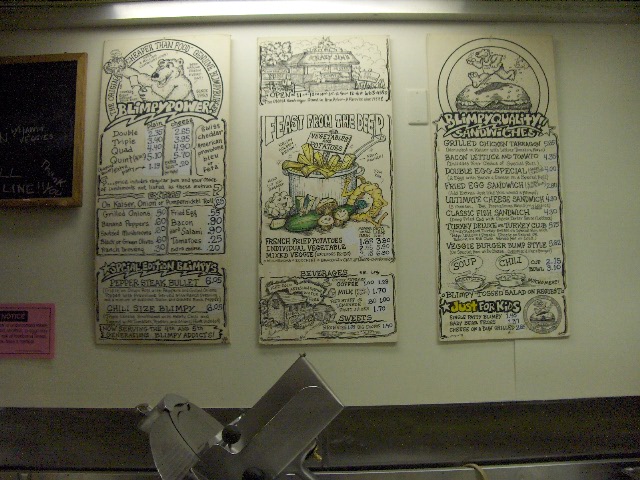The restaurant wall displays three densely packed, hand-drawn menu boards, evoking a charming, old-fashioned vibe. Each board is brimming with an array of menu items written in intricate detail. 

On the leftmost menu, titled "Blimpy Power," a cheerful bear illustration welcomes diners. This section highlights breakfast items such as fried eggs and bacon, alongside various lunch and dinner options. Special mention is given to the "Special Edition Blimpies," including the "Pepper Steak Bullet" priced nostalgically at $6.95, suggesting the menu is from an earlier time.

The central menu, labeled "Feast from the Deep," primarily features seafood dishes complemented by sides like vegetables and potatoes. It also includes a beverages section offering a variety of drink options.

The rightmost menu, titled "Blimpy Quality Sandwiches," lists a range of sandwich options such as grilled chicken. There are also sections dedicated to a double egg special, kids' menu items, and hearty offerings like soup and chili. The overall aesthetic and pricing imply a cozy, historic eatery that focuses on comfort food and family-friendly meals.